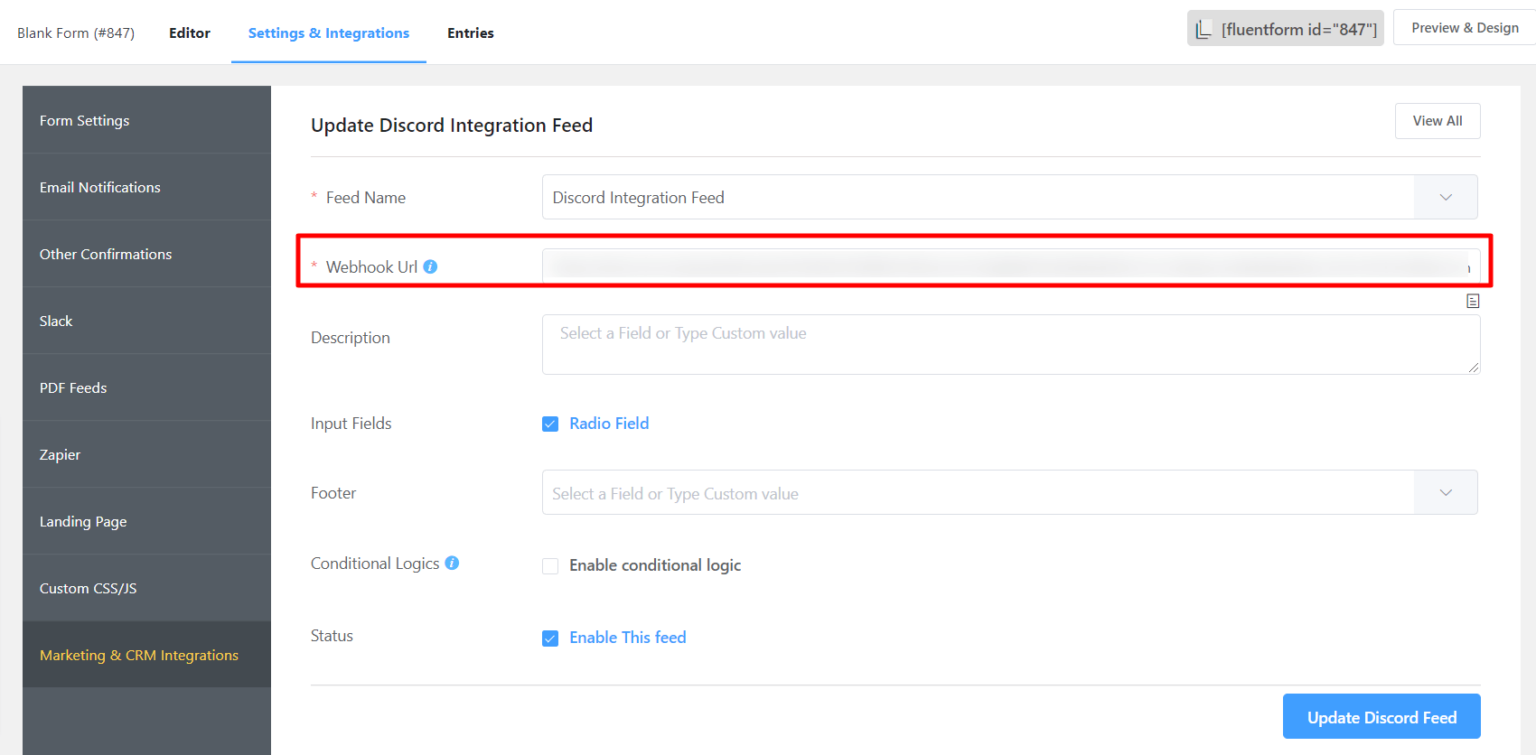The image depicts an extensive administrative dashboard interface meant for managing various integrations and settings. On the left side of the screen, there is a dark grey or slate navigation pane featuring white text, listing options such as "Form Settings," "Email Settings," "Confirmations," "Slack Feeds," "Zapier Integrations," "Landing Page," and "Custom CSS." 

Prominently displayed in the middle of the interface is a section specifically dedicated to Discord integration. This part asks the user to fill out several input fields, including a webhook URL, a description, and other relevant information. Some fields are already checked off, such as a radio field meant to select from multiple options. There's also a footer area, and options to apply conditional logic to the integration.

Towards the bottom right of this admin interface, a blue button labeled "Update Discord Feed" offers the ability to finalize the settings entered. The background of the main page is generally white, emphasizing clean and clear visibility of the tools available for use. This dashboard appears to be designed for mods or administrators who use third-party tools to connect and manage integrations within Discord.